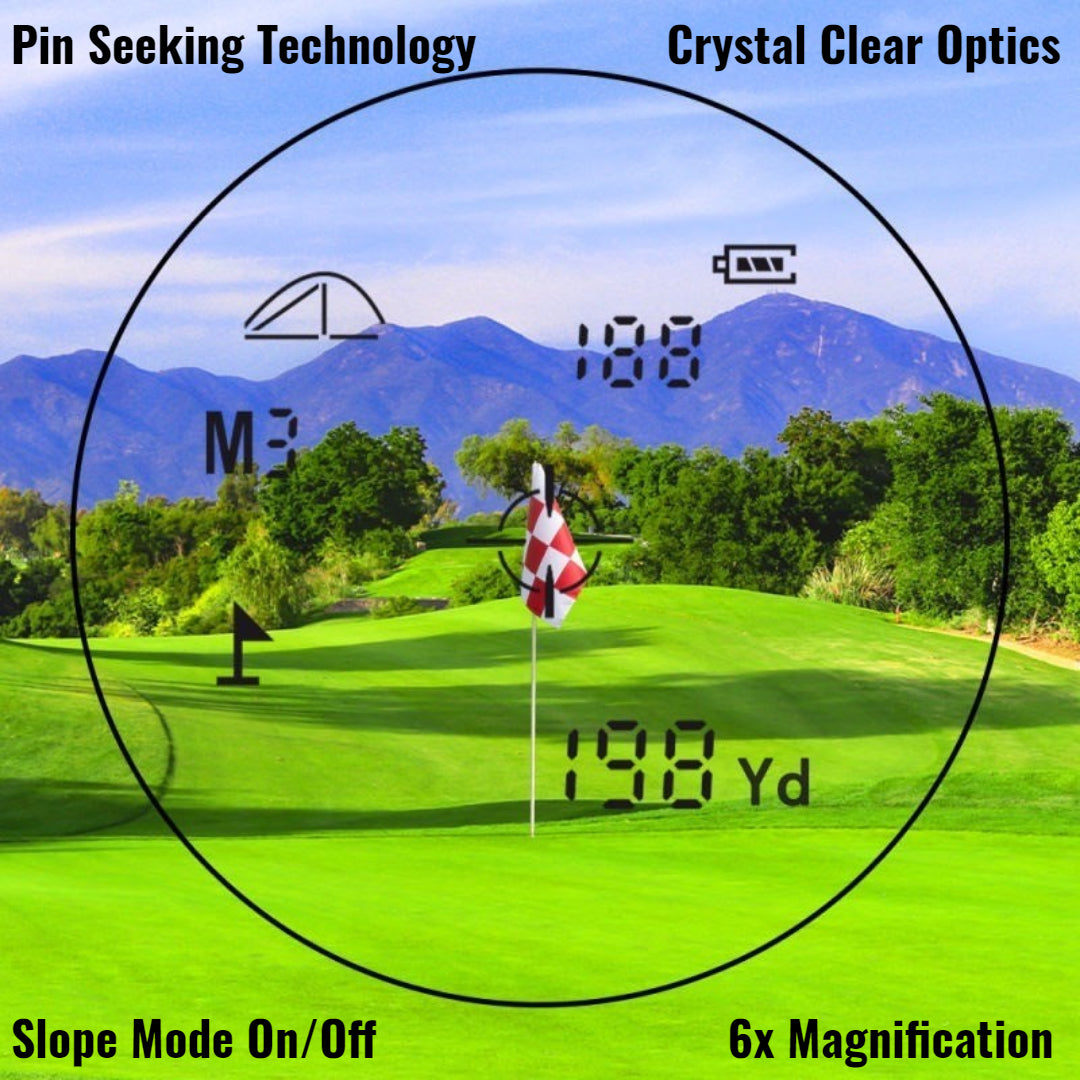This image is an advertisement for a high-tech golf assistant tool, displayed against a vibrant golf course backdrop. Dominated by a lush, well-maintained green, the scene is framed by verdant trees and majestic mountains under a clear blue sky. Central to the image is a red and white checkered flag marking the 198-yard hole, depicted within the crosshairs of this targeting device. Important features are highlighted through various text overlays: "pin-seeking technology" is prominently displayed in the top left corner, while "crystal clear optics" graces the top right. The bottom left corner indicates the availability of "slope mode on/off," and the bottom right confirms the tool’s capability of "6x magnification." A full battery indicator assures users of its readiness. The device also displays a number "188," although its exact significance remains unclear. The shadows cast over the gently sloping fairway add depth and realism to this promotional representation, enhancing the appeal of the product.